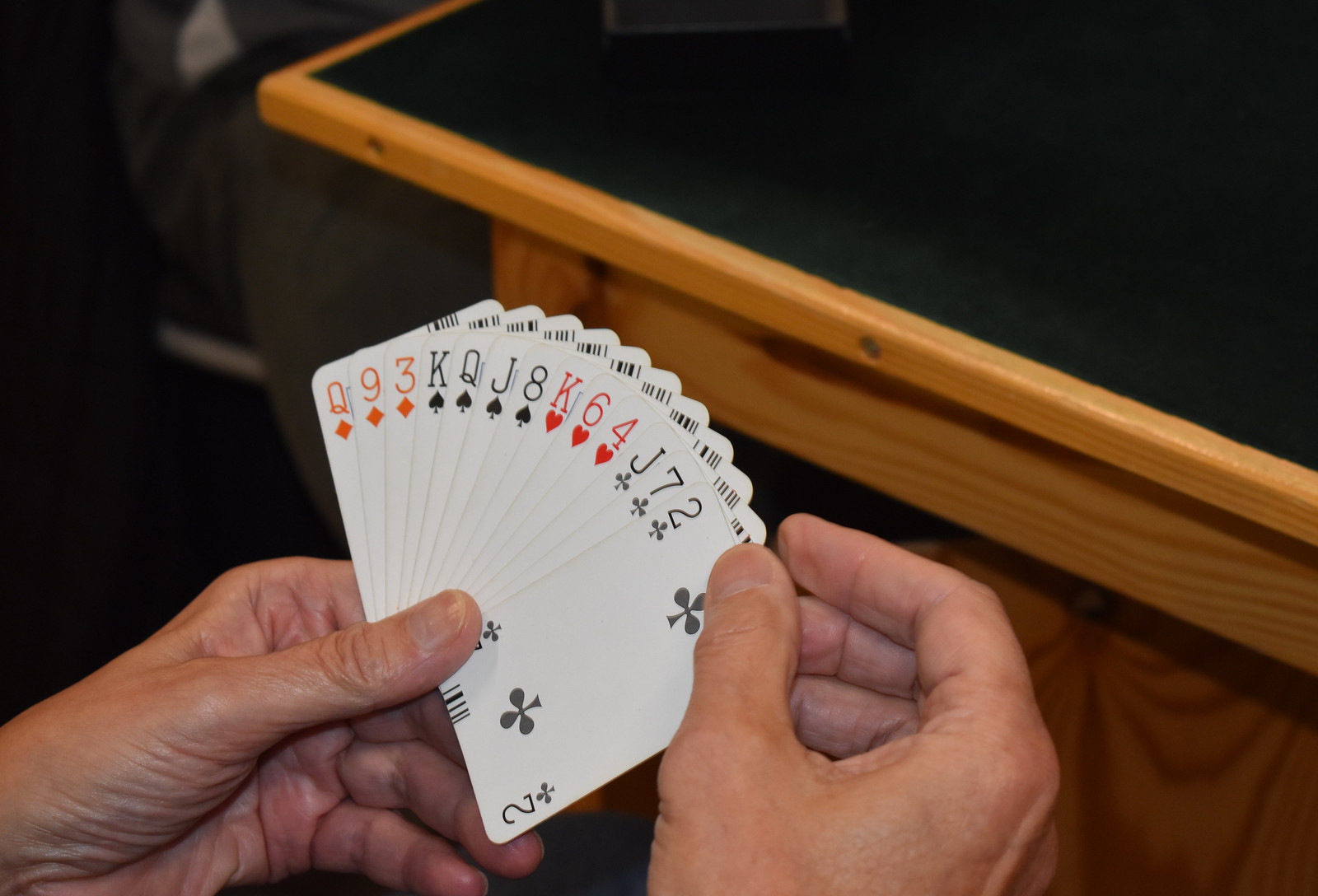This photograph captures an individual holding a fanned hand of playing cards. The cards visible in the hand include the Queen of Diamonds, 9 of Diamonds, 3 of Diamonds, King of Spades, Queen of Spades, Jack of Spades, 8 of Spades, King of Hearts, 6 of Hearts, 4 of Hearts, Jack of Clubs, 7 of Clubs, and 2 of Clubs. The person holds the cards with their left hand, while their right hand is just starting to shuffle through the deck using the tips of their fingers. The scene is set at an all-purpose game table, which is commercial in style and sturdy, with visible screws and strength-enhancing pieces on the sides. The table has a black, multi-purpose surface, and a thick blonde trim along the edges, indicating a robust design suitable for a community center or facility rather than a home game room. In the background, the darkness is complemented by an out-of-focus image of another chair, possibly occupied, hinting that the individual might be engaged in a game with others. The overall focus remains on the cards and the hands, providing a detailed glimpse into the moment of shuffling a dealt hand.